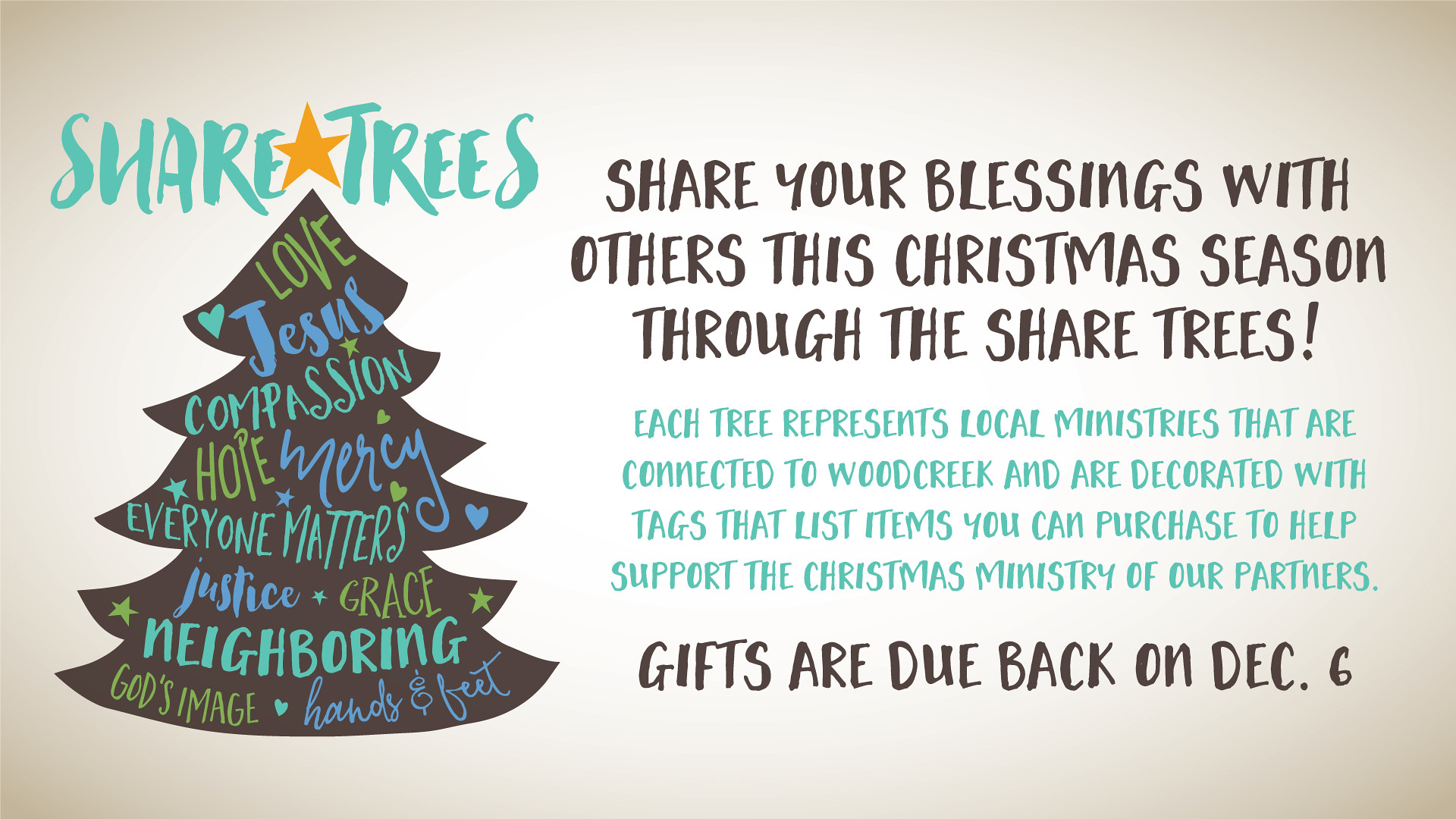This advertisement features a childlike, handwritten design on a beige-ish sepia background, incorporating light greens, browns, and blues. The left side of the graphic prominently displays "Share Trees" in teal text, with a star placed between the words, completing a Christmas tree illustration beneath. The tree itself is adorned with various words in mixed fonts, including "love," "Jesus," "compassion," "hope," "mercy," "everyone matters," "justice," "grace," "neighboring," "God's image," and "hands and feet." 

To the right, in black text, it reads: "Share your blessings with others this Christmas season through the Share Trees!" and further explains in smaller teal text, "Each tree represents local ministries connected to Wood Creek and is decorated with tags listing items you can purchase to support our partners' Christmas ministry." Below that, a note in black text emphasizes that gifts are due back on December 6th.